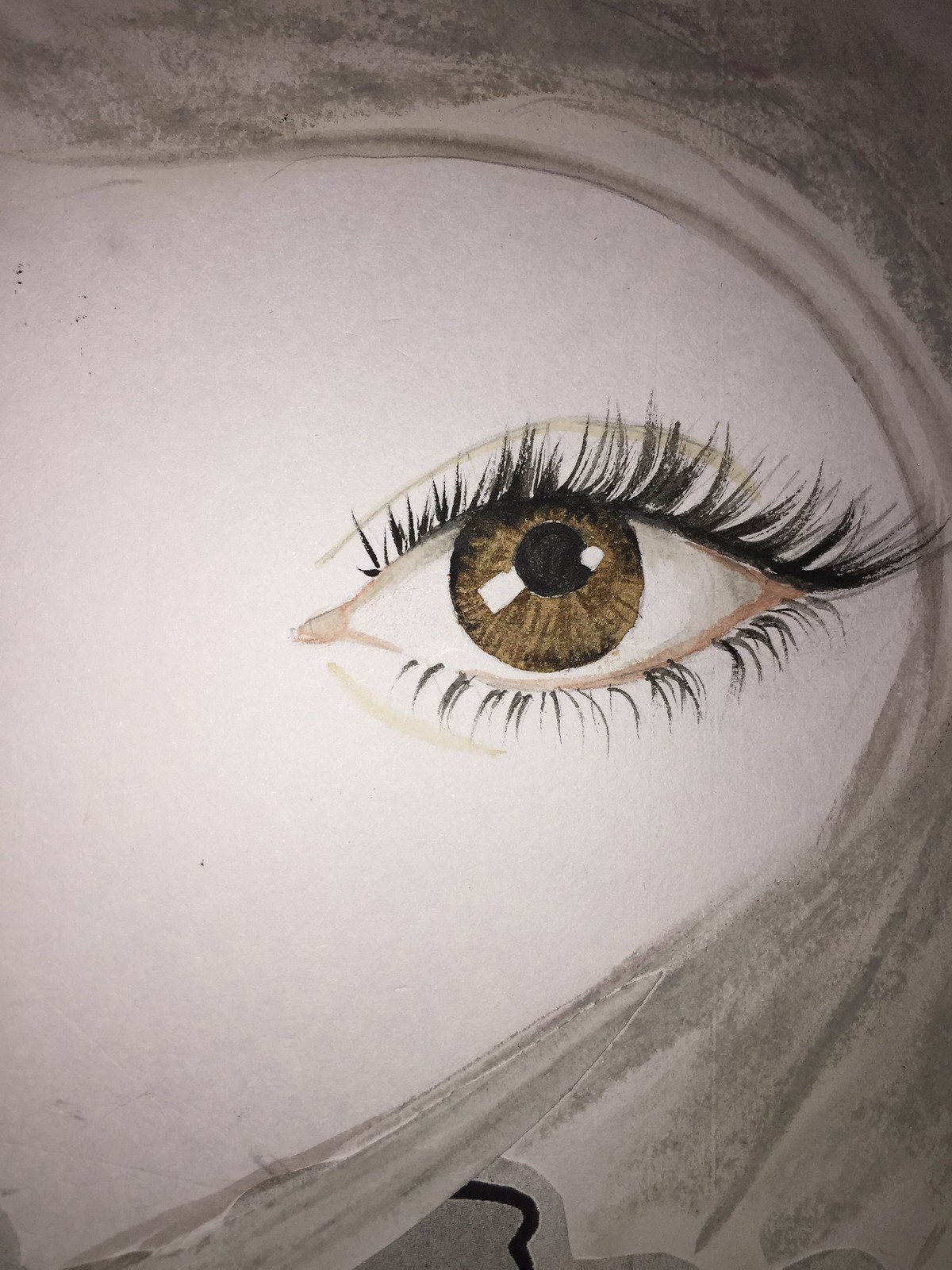The image is a highly detailed, realistic drawing of a single human eye, prominently displayed toward the center of the portrait-oriented sketch. The eye, characterized by its brown iris with intricate striations and black specks, exhibits a masterful depiction of light reflections on both sides of the pupil. The detailing is so refined that the eyelashes, both upper and lower, appear almost tangible, reminiscent of real or even false lashes. The white conjunctiva and the slight pink hue add a touch of realism, as does the subtle shadowing below the eye and near the eyelid crease. Surrounding the eye is a soft, velvet-like texture with gray shading, possibly suggesting a scarf or head covering draped around the face, though no other facial features like the nose or the other eye are visible. The overall composition suggests a left eye, with its meticulous details and shading creating a captivating and lifelike image.